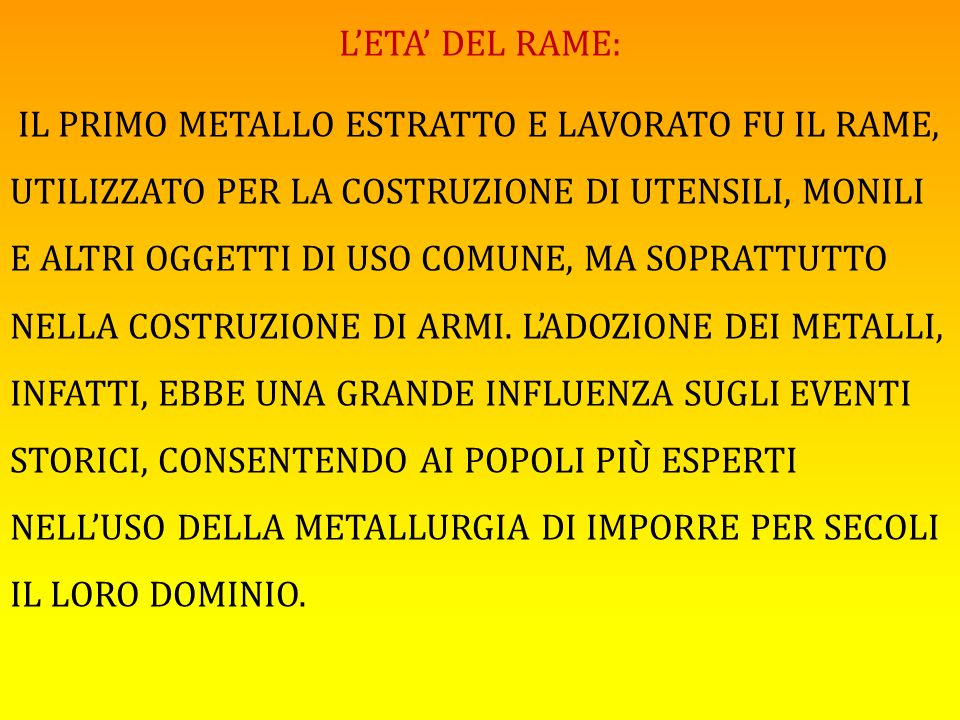The image is a square-shaped PowerPoint or Google slide with a gradient background transitioning from burnt orange at the top to bright yellow at the bottom. The text, written in Italian, begins with "L'ETA DEL RAME" prominently displayed in red, all caps at the top. Below, a large block of text spans almost the entire slide, written in black, all caps, describing the historical significance of copper as the first metal extracted and its applications in utensils, common objects, and, most notably, military weapons. The description highlights how the use of copper influenced historical battles and helped secure dominions. The color palette includes shades of red, orange, yellow, and black, with the text laid out horizontally over the vibrant background.